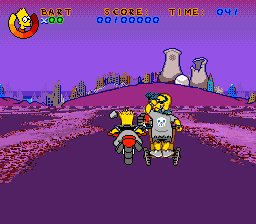This image is a screenshot from a video game based on The Simpsons. Dominating the scene is a dark purple road that winds through a cartoon city sitting on a light purple hill with a nuclear power plant visible in the distance. The road is lined with small purple flowers, adding a whimsical touch. In the foreground, Bart Simpson can be seen from behind, riding a motorcycle with red accents and large tires, while Homer Simpson is on a smaller, two-wheeled vehicle. Both characters are shown with their distinctive yellow skin. In the upper left-hand corner of the screen, there is a profile picture of Bart Simpson, accompanied by 'Bart' and 'X00' text. Next to it, the score is displayed in blue as '100,000' and the remaining time is shown as '41'. The background and overall aesthetic feature vibrant, cartoony colors, staying true to The Simpsons' iconic style.